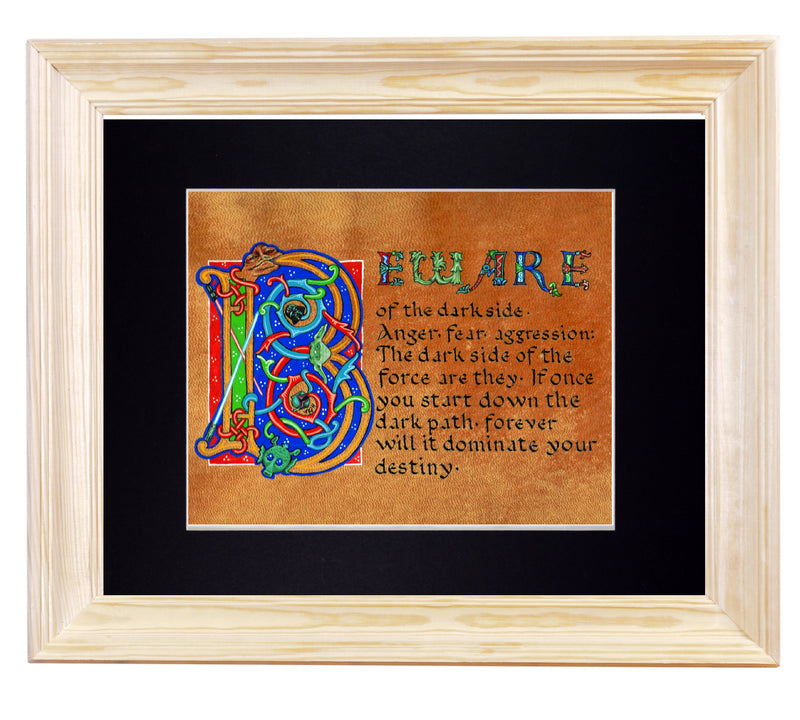This image features a square picture frame made of light wood with slightly darker grains running through it. The frame is thick and contrasts against a white background. Inside the frame, the backing is solid black, and against this backdrop sits a vibrant orange square. Dominating the center of the square is a large, multicolored letter "B" formed by swirling lines in blue, orange, green, and red. To the right of this ornate "B," the letters "E-W-A-R-E" appear in smaller multicolored text, collectively spelling out "Beware." Below this, in black text, it reads: "of the dark side, anger, fear, aggression, the dark side of the Force, are they? If once you start down the dark path, forever will it dominate your destiny." The artwork within the frame conveys a message that echoes the wise words of Yoda, enriched with a medieval art style and surrounded by a black thick border.